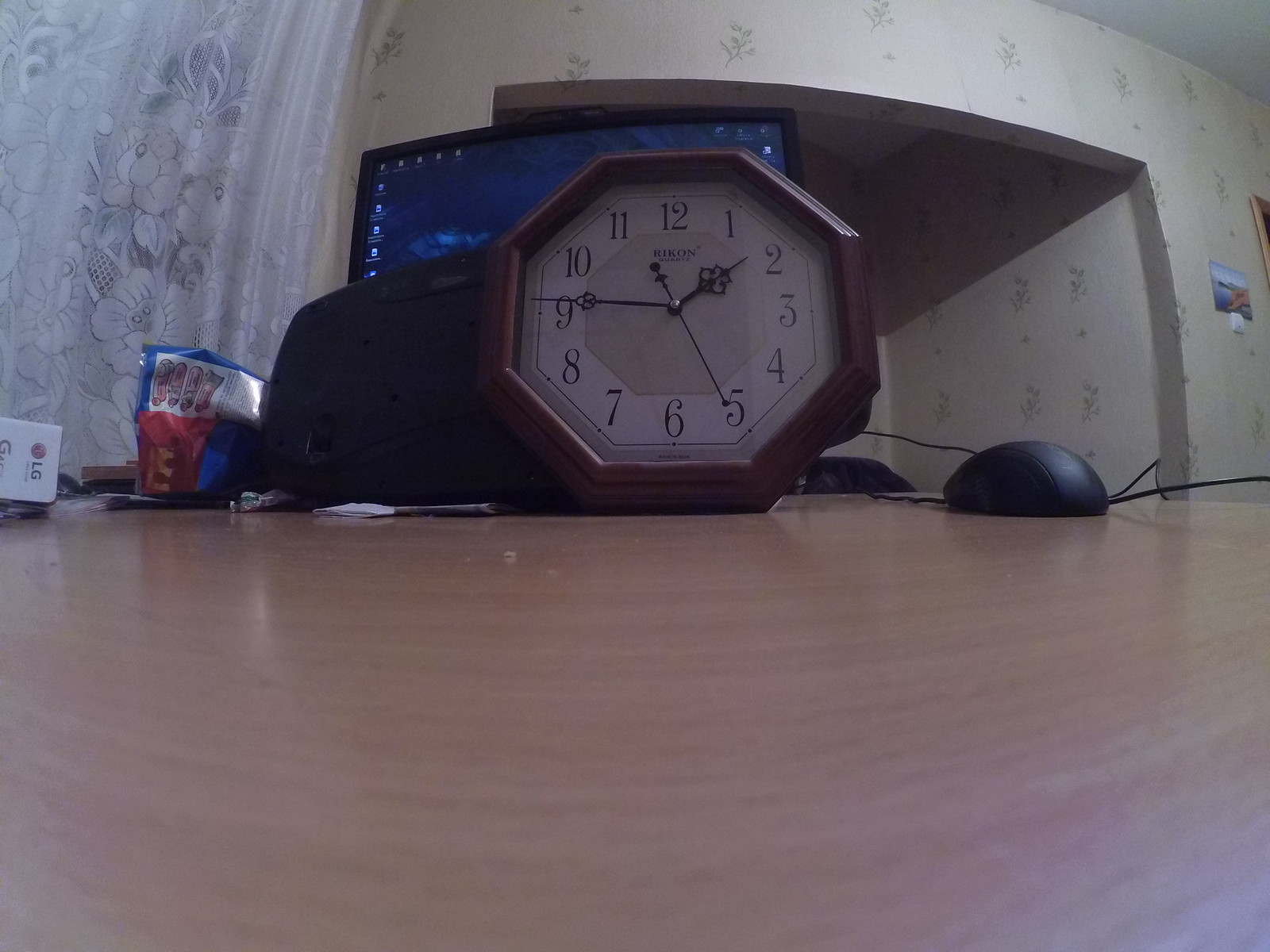In this photograph, a wall clock is prominently featured, though intriguingly it is resting on a light oak-colored wooden table rather than being mounted on a wall. The clock's face is white, with bold black numbers ranging from 1 to 12, and it is encased in a wooden brown border. The time displayed on the clock is 1:47 and 25 seconds. Positioned near the clock is a black computer mouse, also on the table. Behind the clock, a computer monitor is visible, displaying an active program. To the left of the scene, a few indistinct child's toys can be seen adding a touch of whimsy to the setting.